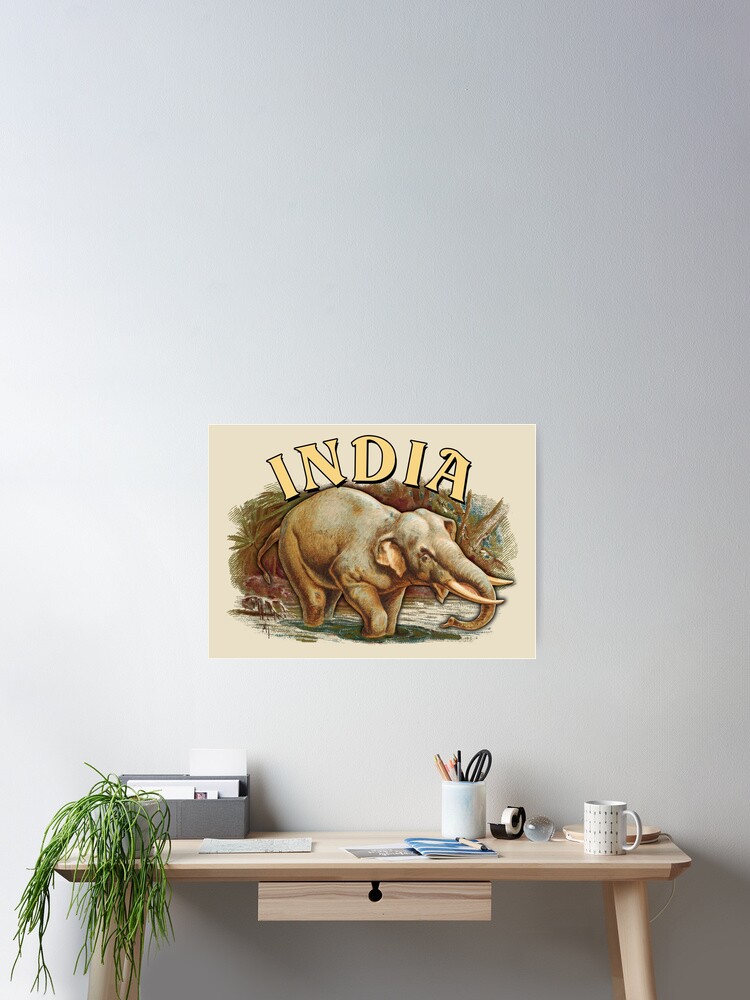The image depicts a simple indoor setting featuring a light wooden desk positioned against a soft gray wall that gradually lightens towards the bottom left. The wall is adorned with a poster displaying the word "India" in bold yellow letters above an illustration of an elephant trudging through water. The desk itself has four legs that slightly splay outwards and includes a small central drawer with a minimalistic handle.

On the desk, a white, bendable desk lamp with a visible wire is positioned towards the right side. To the left, there's a small spider plant whose cascading branches add a touch of greenery to the scene. Adjacent to the plant is a gray file container. The desktop also features a white mug containing scissors and various writing implements, a tape dispenser, and a coffee mug. The overall arrangement is both functional and aesthetically simple, highlighting the desk as the focal point within the softly lit room.